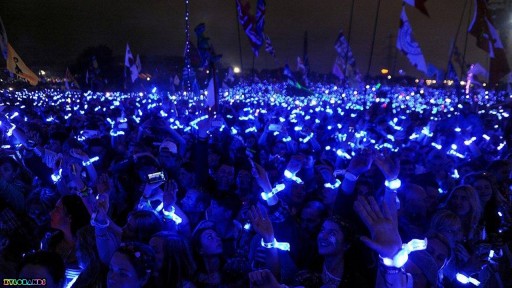In the image, a large, nighttime gathering of people stretches off into the horizon, bathed in a light blue glow from their glow-in-the-dark wristbands and watches. The crowd, predominantly composed of women, raises their arms, illuminating the scene with their blue-themed light. The setting appears to be outdoors, perhaps for a concert, rally, or significant event. In the background, numerous flags of various colors—including black, white, and blue—are held high on poles, though their details are indistinct. The sea of glowing wristbands extends far back, creating a mesmerizing effect that fills the entire photo with a unifying luminescence.